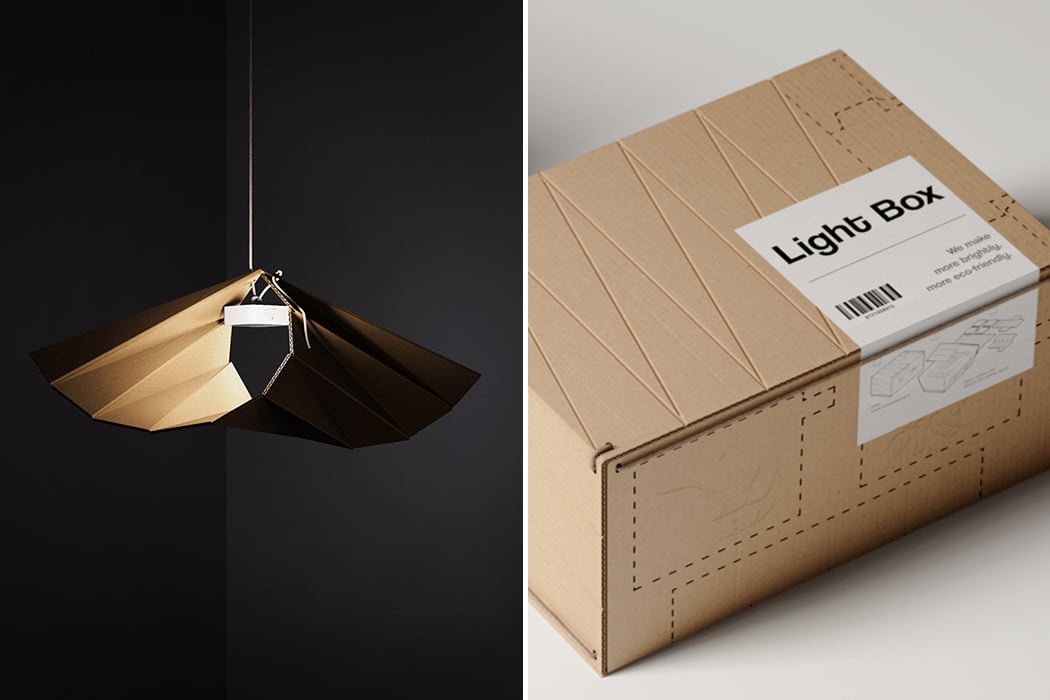The image features two photographs displayed side by side. The left photograph showcases a uniquely designed, hanging pendant light fixture, constructed from louvered cardboard. The light device, which resembles the shape of a mustache, is brown in color and hangs from a contrasting white cord against a background of gray and darker gray walls. Notably, the actual light bulb is obscured, emphasizing the artistic structure of the fixture.

On the right, there is an unopened rectangular cardboard box placed against a grayish-white background. The box features a prominent white label that reads "Light Box" with additional gray lettering underneath stating, "we make more brightly, more eco-friendly." The label also includes a UPC barcode and a diagram illustrating the assembly instructions for the light fixture. The perforation dots on the box indicate where to cut for opening. The combined visual information of the two images shows the boxed light kit on the right and its assembled form on the left.